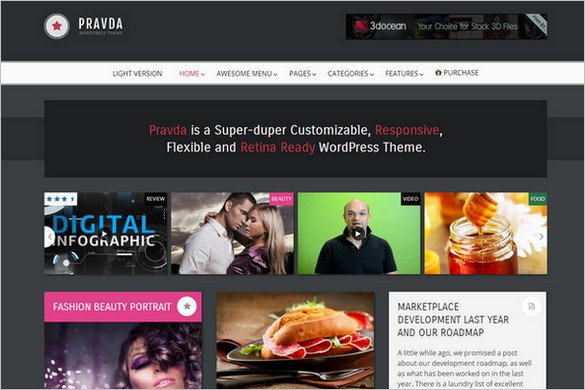This image, sourced from the website PRAVDA, features a detailed layout and design. In the upper left corner, there's a prominent white circle with a red star, representing the site's logo. On the upper right-hand side, a small banner displays the text "Your choice for stock 30 files." 

Immediately below this banner, a horizontal white navigation bar spans the width of the page. The menu options, listed from left to right, include "Light Version," "Home," "Awesome Menu," "Pages," "Categories," "Features," and "Purchase." 

Beneath this navigation bar, a square box contains the text: "Pravda is a super-duper customizable, responsive, flexible and retina-ready WordPress theme."

Further down, the layout divides into four distinct blocks. The first block showcases a digital infographic. The second block features an image of two people standing chest-to-chest. The third block appears as a video thumbnail of a person speaking. The fourth and final block displays an image of a jar of honey.